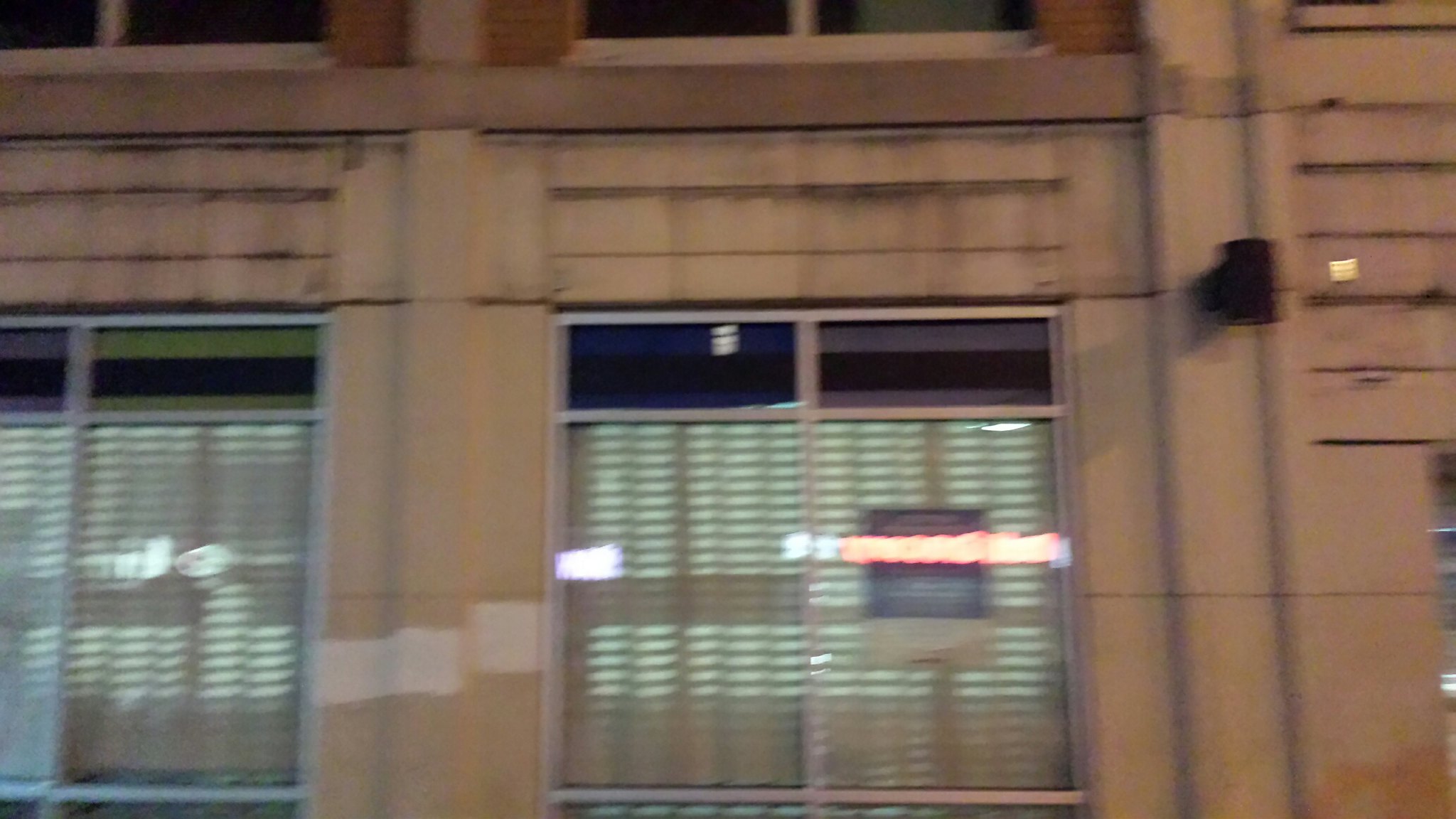This photograph captures the side of a multistory building, likely made of brownish concrete with a textured surface, taken at an eye-level perspective from the sidewalk or just off the street. Dominating the middle of the image, there are two square windows aligned side by side, adorned with metal frames that divide each window into four smaller rectangles. A significant feature between these windows is a squared-off section extending outward from the flat facade.

The windows feature closed blinds, with slight light seepage and reflection occurring, particularly noticeable in the right window that bears a white sticker on the inside. The reflecting neon light seen in the window is likely from a sign across the street, specifically a blue rectangular sign on a pole. Further enhancing the intricate detail, silver trim surrounds the windows, and above them, there are decorative borders: one with green-black-green and another with blue-black-blue color schemes.

The top of the photo shows the lower segments of two more windows with brown shutters and white seals, partially visible and hinting at additional stories above. The building's surface showcases elements of painted brickwork above each window, contributing to a complex and captivating aesthetic.